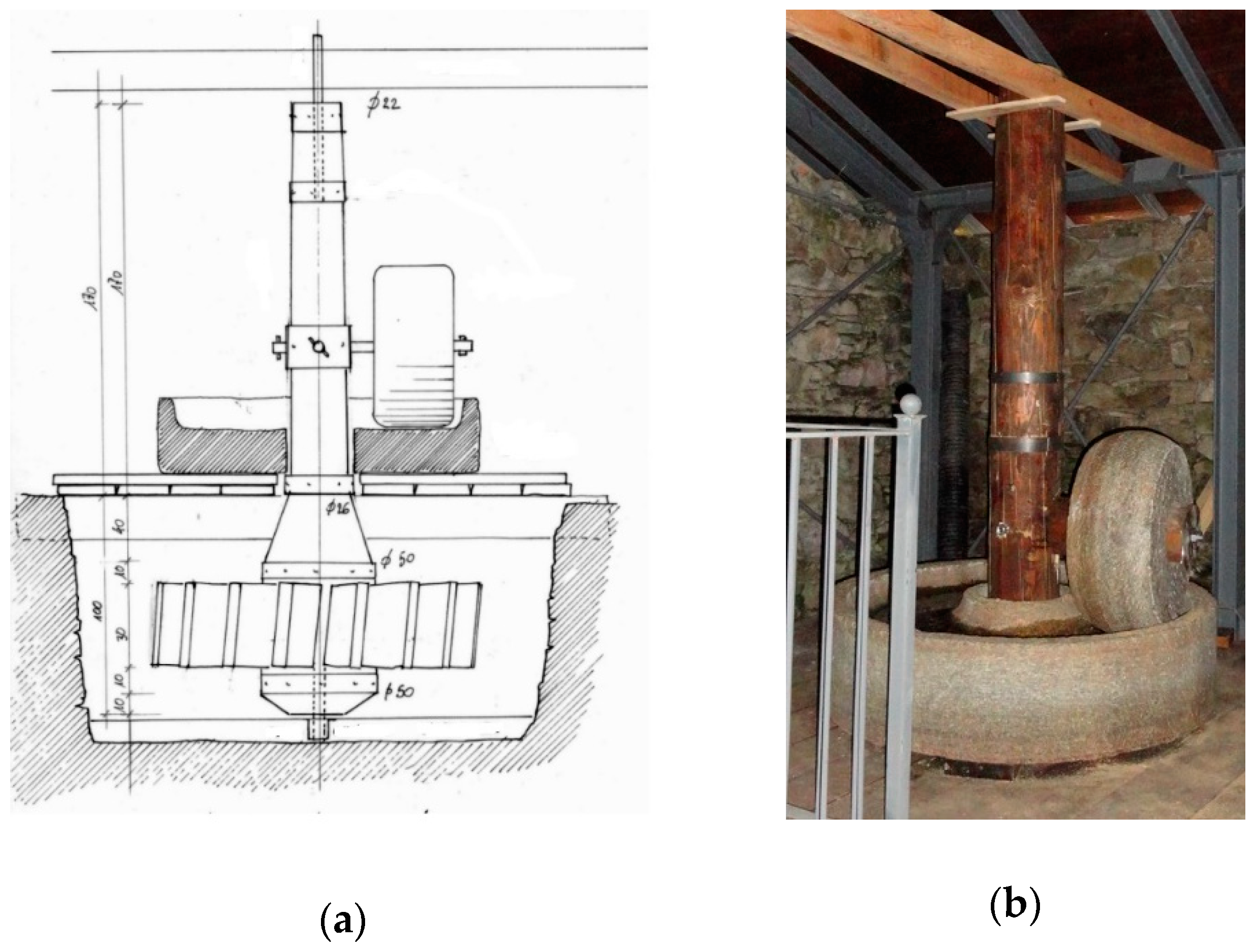The image features two side-by-side sections labeled A and B. section A, on the left, is a detailed black and white blueprint depicting some sort of drilling equipment or septic system, with intricate designs suggesting a complex mechanism. On the right, section B is a color photograph providing a realistic view of the equipment. The photograph shows a basement with a clean, cement floor, brick walls, and a black ceiling supported by wooden beams extending from both ends. The focal point in section B is a prominent wooden pole planted in the center, protruding into a circular stone base. Atop this base lies a smaller, gray circular stone placed sideways. The blueprint in section A visually aligns with the real-life setup in section B, indicating that section A is the design plan for the equipment shown in section B.